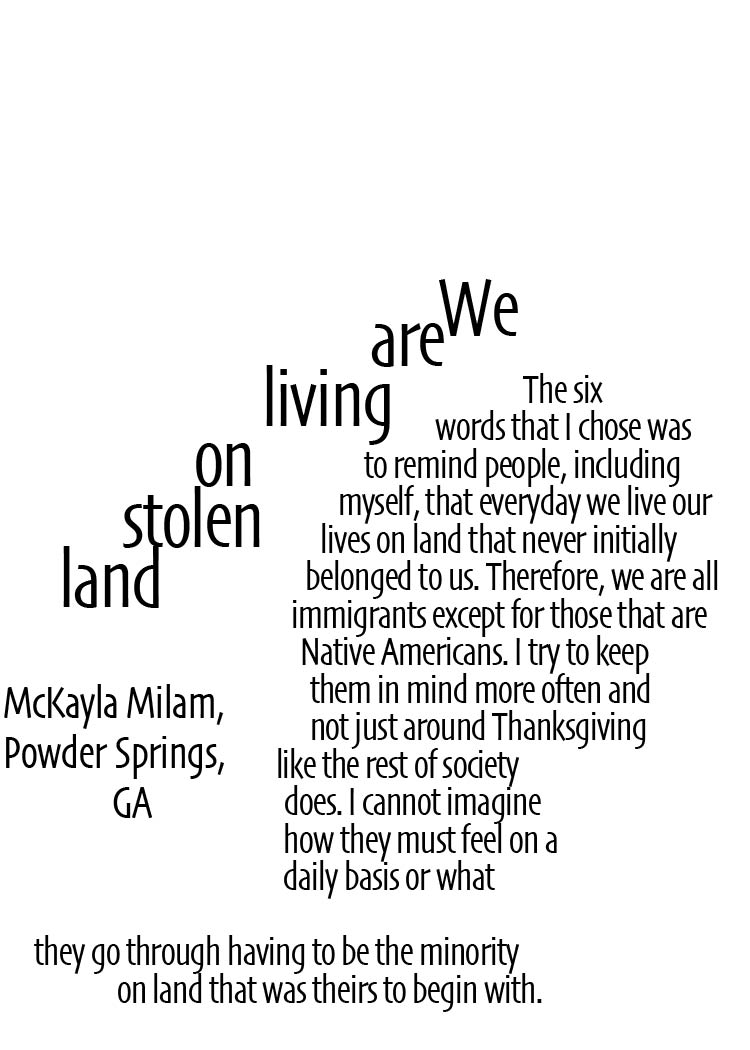The image features an artistic arrangement of text on a white background with black lettering. On the left side of the image, one word per line, slanting downward, reads: "We are living on stolen land." Below this vertical text, the author, Michaela Milam from Powder Springs, Georgia, is credited. On the right side of the image, a paragraph expands upon the central theme. It states that the phrase "We are living on stolen land" serves as a reminder, to the author and others, that the land we live on was not originally ours and that, except for Native Americans, we are all immigrants. The author emphasizes the importance of remembering Native Americans' experience and struggles not just during Thanksgiving, as is common, but throughout the year. They reflect on the daily hardships endured by Native Americans, who are now a minority on what was once their own land.